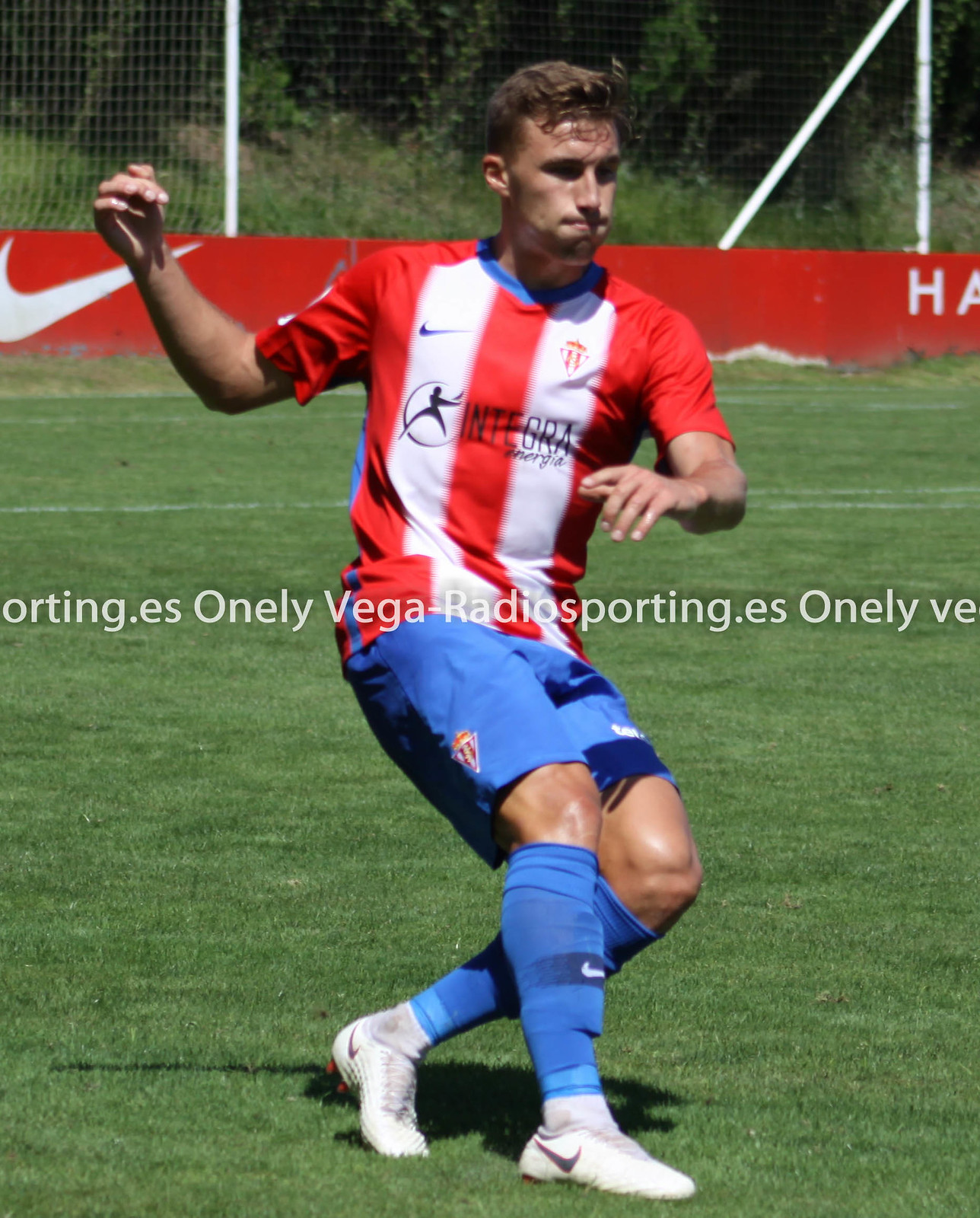The photograph captures a dedicated soccer player mid-action on the field. He is outfitted in a distinctive red and white vertical-striped shirt with a blue collar, branded with the Nike logo and the name "Integra." His uniform extends to blue shorts, complemented by blue socks and white Nike shoes. The player also sports blue knee guards and shin pads, all of which prominently display the Nike logo. He leans back, one leg folded behind him and his right arm raised, showcasing his intense concentration. His curly hair is matted with sweat, reflecting the exertion of the game. The green grass of the soccer field is evident, with netting visible in the background, and a soccer banner featuring a large white Nike logo and partially obscured text. Across the image, a watermark reading "OnlyVegaRadioSporting.es" repeats in a pattern.